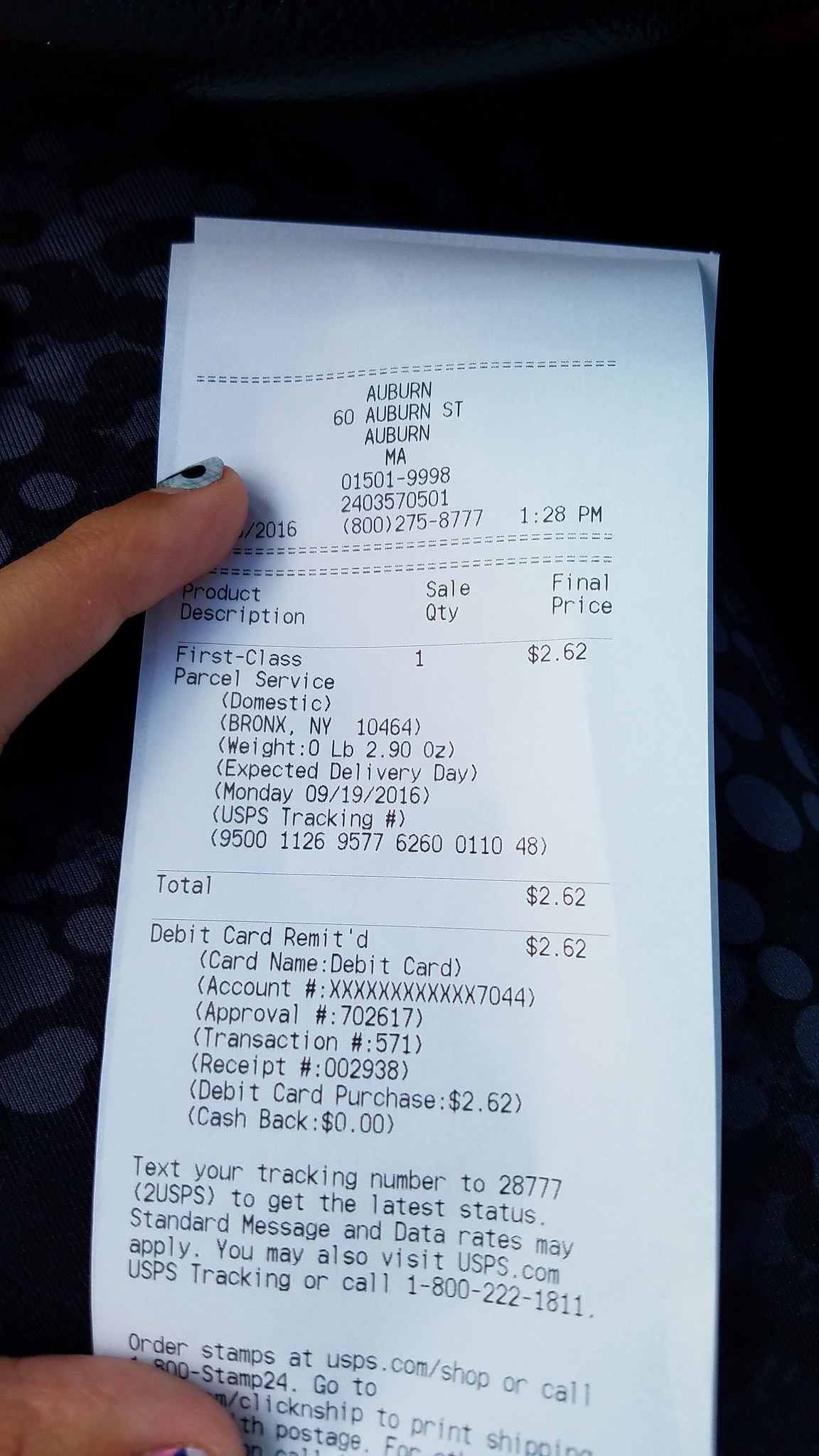The image features a detailed United States Postal Service (USPS) receipt being held flat by an individual's left hand to prevent it from curling up. The person's thumb is positioned at the bottom and their index finger at the top of the receipt. The transaction took place at a USPS location in Auburn, situated at 60 Auburn Street, Auburn, Massachusetts. The receipt lists the relevant phone number, along with the transaction's date and time.

This specific purchase included a First Class Parcel Service for a package weighing 2.9 ounces, destined for the Bronx, New York, with an expected delivery date of Monday, September 19, 2016. The final price for this service was $2.62. The receipt also displays key details such as the USPS tracking number, last four digits of the debit card used for payment, and various transaction identifiers like receipt number and approval code. Additionally, it suggests that the customer can text their tracking number to receive the latest status updates on their package.